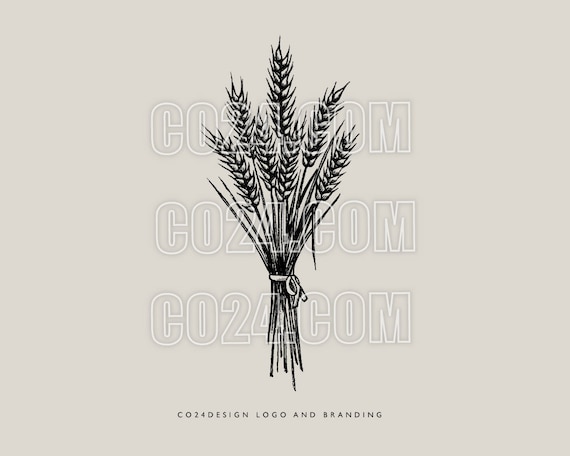This black and white illustration depicts a bundled sheaf of wheat, tied together with a ribbon in a hand-drawn style. The bundle, consisting of six to eight stalks with full wheat heads at the top, is centrally positioned on a light gray background. Superimposed on the wheat image is the opaque text "CO24.com," highlighted with a white trim. At the bottom of the illustration, it reads "CO24 Design Logo and Branding" in black text. The overall design appears to be a logo sample, demonstrating the company's branding capabilities, with the "CO24.com" text repeated three times as a watermark to prevent misuse.